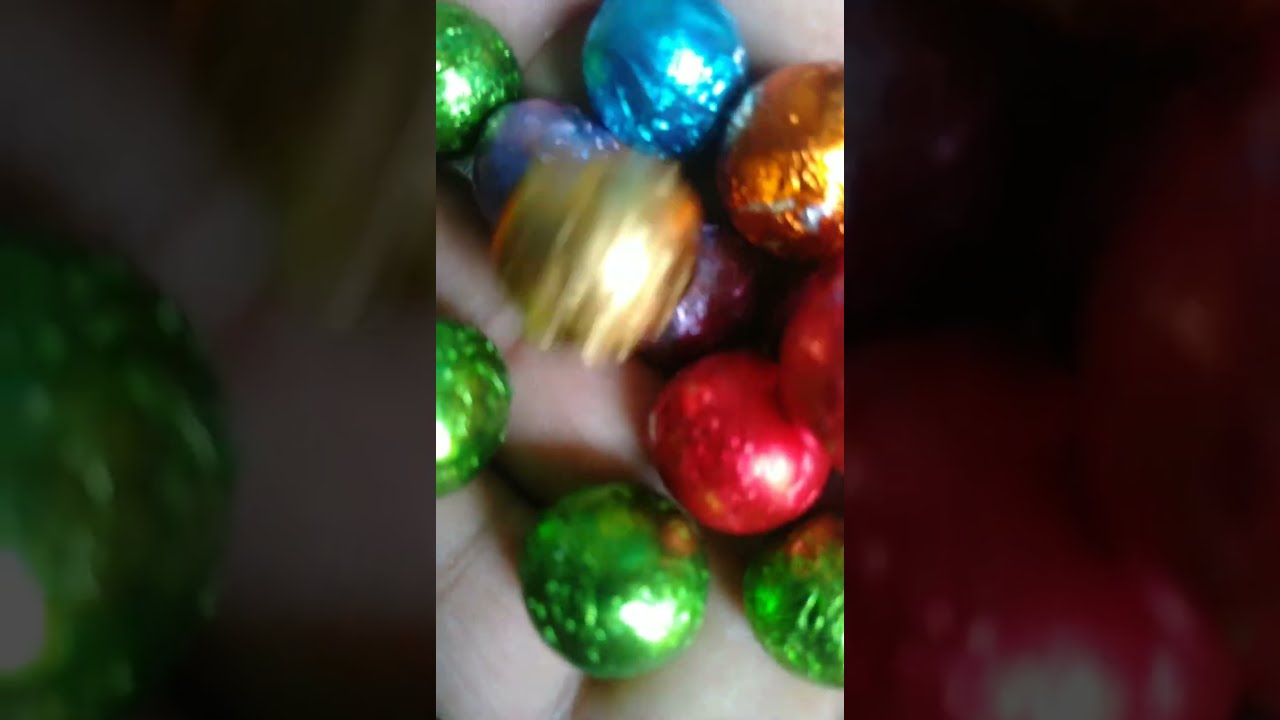The image is a vertical cell phone photograph featuring a collection of shiny, multicolored spherical ornaments, which could be Christmas decorations or candy balls with a metallic wrapping. The main image is centered, with faded, zoomed-in sections on either side, providing an expanded but less distinct view of the same scene. The ornaments rest on a gray surface, possibly a hand, and are illuminated by a light source that causes bright reflections on their surfaces. Colors include green, red, blue, purple, gold, and dark orange, with the gold one appearing in motion above the rest, creating a motion blur effect. Notably, the gold ornament near the center is out of focus and seems to have streaks of light, adding to its dynamic appearance. Overall, the setting gives a festive and shiny appearance with a mix of in-focus and blurred elements, enhancing the visual appeal.